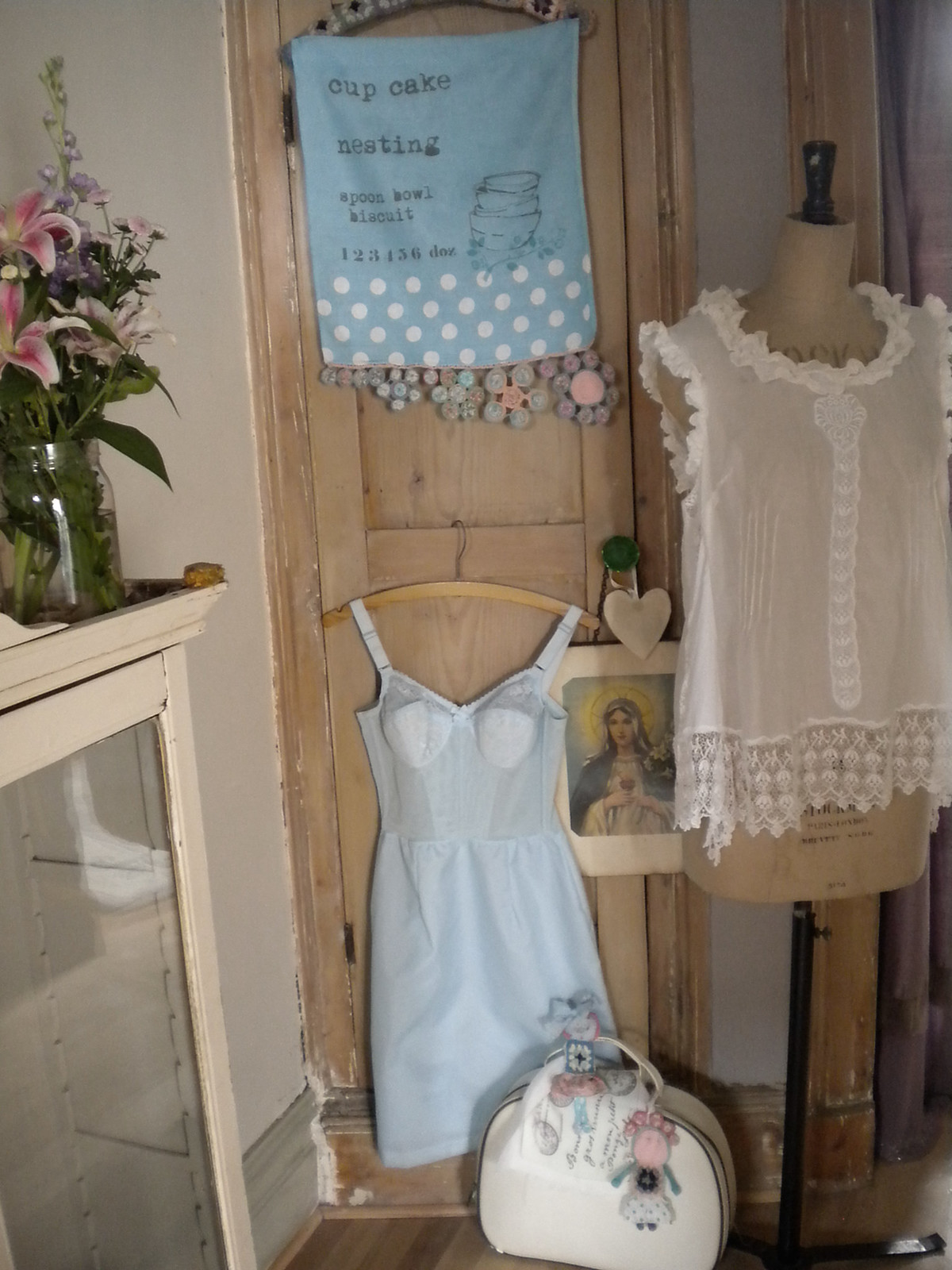The image captures a detailed view of a room featuring a wooden door with multiple items arranged thoughtfully. On the right side, there's a half mannequin dressed in a sheer, sleeveless white lace blouse with frilly details on the neck and shoulders. In front of the door, there’s a light blue dress and a white bag placed on the floor, with a pink doll-like accessory hanging from the bag. The left side of the composition showcases a jar used as a vase, filled with pink flowers atop a drawer.

Hanging on the door is a towel adorned with the words “Cupcake,” “Nesting,” “Spoon,” “Bowl,” “Biscuit,” and the numbers “1, 2, 3, 4, 5, 6.” The towel also features an illustration of bowls stacked on top of one another. Above these elements, there is an image of Saint Mary, adding a spiritual touch to the scene. The setting appears to be inside a wooden closet or armoire, suggesting a cozy, eclectic, and meticulously arranged space.